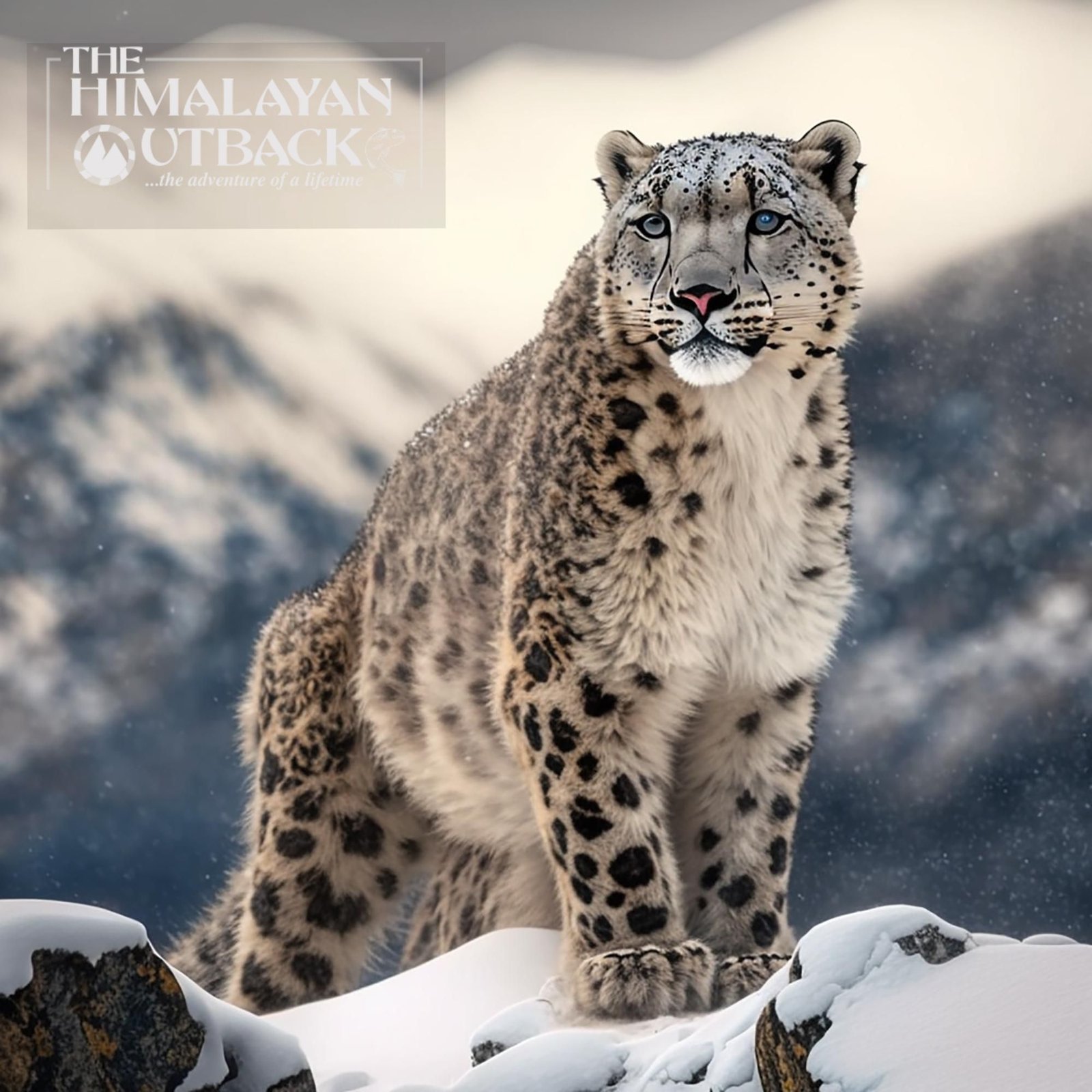The image captures a breathtaking scene of a snow leopard, a large feline predator, standing majestically on snow-covered rocky terrain. His luxurious, thick fur, which is predominantly tannish-white with distinctive black spots, catches the light. His impressively long tail trails behind him, and his big paws are dusted with snow. The snow leopard’s captivating blue-gray eyes peer into the distance, beneath a small pair of ears that sit atop his head. His black nose, accented with a patch of pink, and prominent whiskers complete his regal visage. In the hazy background, jagged mountain ranges loom, partially blanketed in snow, adding depth and grandeur to the scene. Flakes of snow are falling gently, enhancing the wintry atmosphere. Nestled in the upper left-hand corner of the image is a text box reading, "The Himalayan Outback," followed by "The Adventure of a Lifetime..." The text features a clear background with a white border and a subtle mountain icon, blending seamlessly with the image’s snowy expanse. This striking photograph brilliantly showcases the serene natural beauty and strength of the snow leopard in its mountainous habitat.